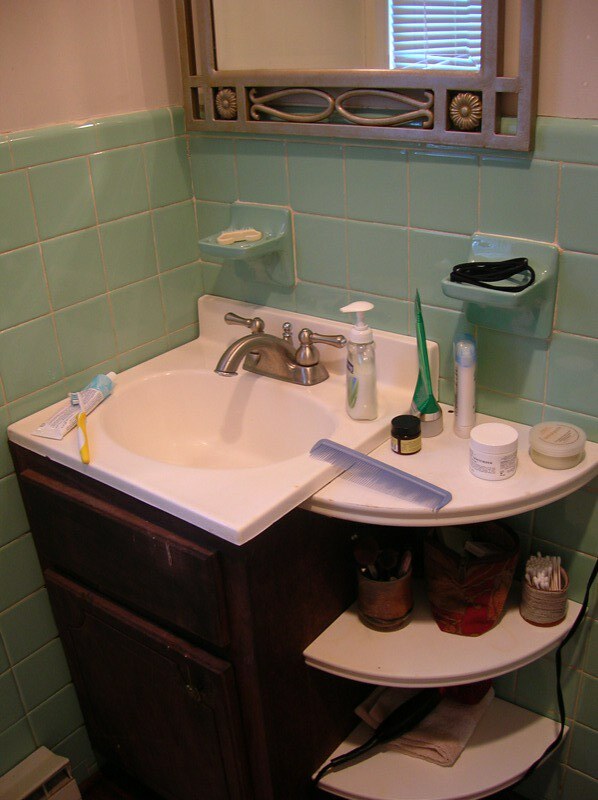In this detailed bathroom photograph, a pristine white ceramic sink is the focal point, adorned with a sleek silver metal faucet equipped with levers on each side for hot and cold water control. A bottle of white-colored hand soap with a blue and green label sits on the right side of the sink, featuring a white pump at the top, although the label is turned away from view. To the left of the sink, a tube of toothpaste lies logo-side down next to a yellow toothbrush.

Underneath the sink, a cabinet made of rich cherry wood showcases a singular drawer above a door, offering a touch of elegance. The sink is set against a vibrant aquamarine tile backsplash that extends to the side wall, creating a striking contrast against the brown wooden framed mirror that hangs above. Inlaid within the tiled wall are two soap dishes of matching aquamarine hue; one holds what appears to be a black hairband, while the other contains a bar of soap.

In the corner, three white corner shelves with rounded fronts and square corners at the back house a variety of products, reflecting practical organization. The shelves display items such as a container of Q-tips, a hairdryer, neatly folded towels, deodorant, and various skincare products, all combining to create a functional and aesthetically pleasing bathroom space.